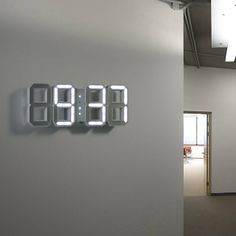The image depicts an interior scene within a building, captured in color and slightly taller than it is wide. The main focus is on a metallic gray wall positioned towards the left side of the picture, adorned solely with a digital clock. The clock lacks a casing, displaying the time 9:37 with its neon white LED digits. The first digit is not illuminated, as it is not needed. Adjacent to this wall, deeper into the image, there is another white wall with an open doorway on its left side, offering a glimpse into a brightly lit room bathed in sunlight. The scene is subtly lit by a fluorescent light located at the top right corner of the image, while the floor in the bottom right appears to be a tan or brown color. This carefully composed photograph captures both the structured simplicity of the clock on the gray wall and the inviting brightness of the adjacent room.